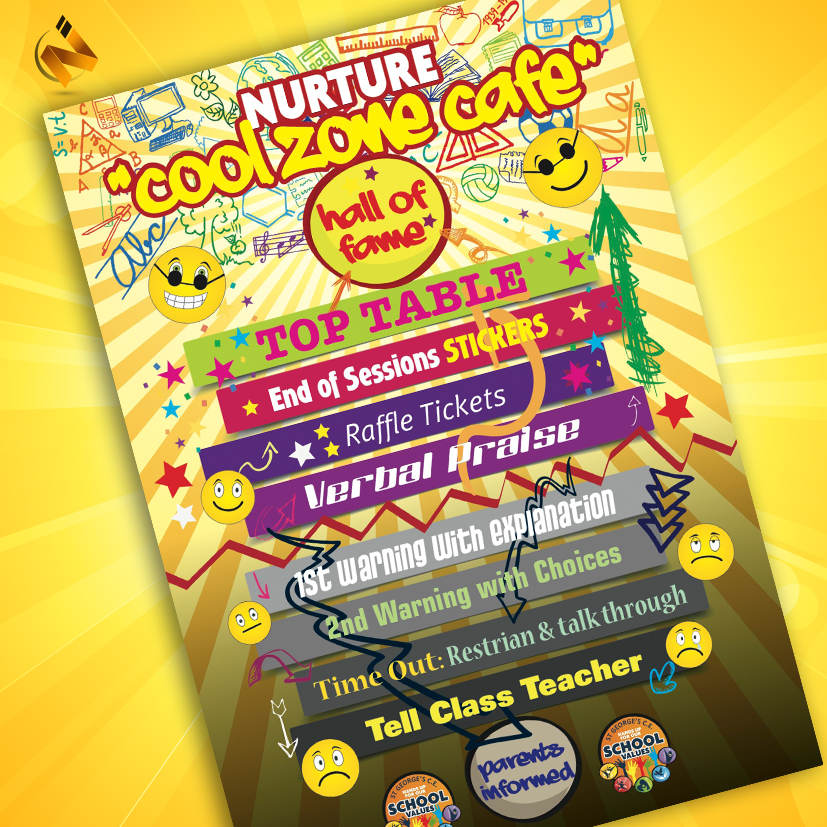The image features a vibrant, yellow school poster titled "Nurture Cool Zone Cafe Hall of Fame," positioned at an angle in the center. This eye-catching poster is adorned with various colorful elements, including a series of distinct banners, each highlighting different levels or activities. The green banner with pink writing reads "Top Table," followed by a pink banner with "End of Sessions Stickers" in white and yellow text. A purple banner with white writing says "Raffle Tickets," while a lighter purple banner also in white text denotes "Verbal Praise." The sequence continues with a light gray banner labeled "First Warning with Explanation" in white, a darker gray banner with green text saying "Second Warning with Choices," and another darker gray banner in yellow and turquoise stating "Time Out, Restrain, and Talk Through." The final banner, a dark gray one with yellow writing, instructs to "Tell Class Teacher," followed by an emphasis on "Parents Informed" at the bottom. Surrounding the text are playful doodles and designs, including a sunburst, various school-related items like a globe, computer, calculator, apple, volleyball, and musical notes, and multiple emojis displaying different expressions, both happy and sad, adding to the poster's lively and engaging appeal. The poster also emphasizes the school's values, marked as "St. George's CE."